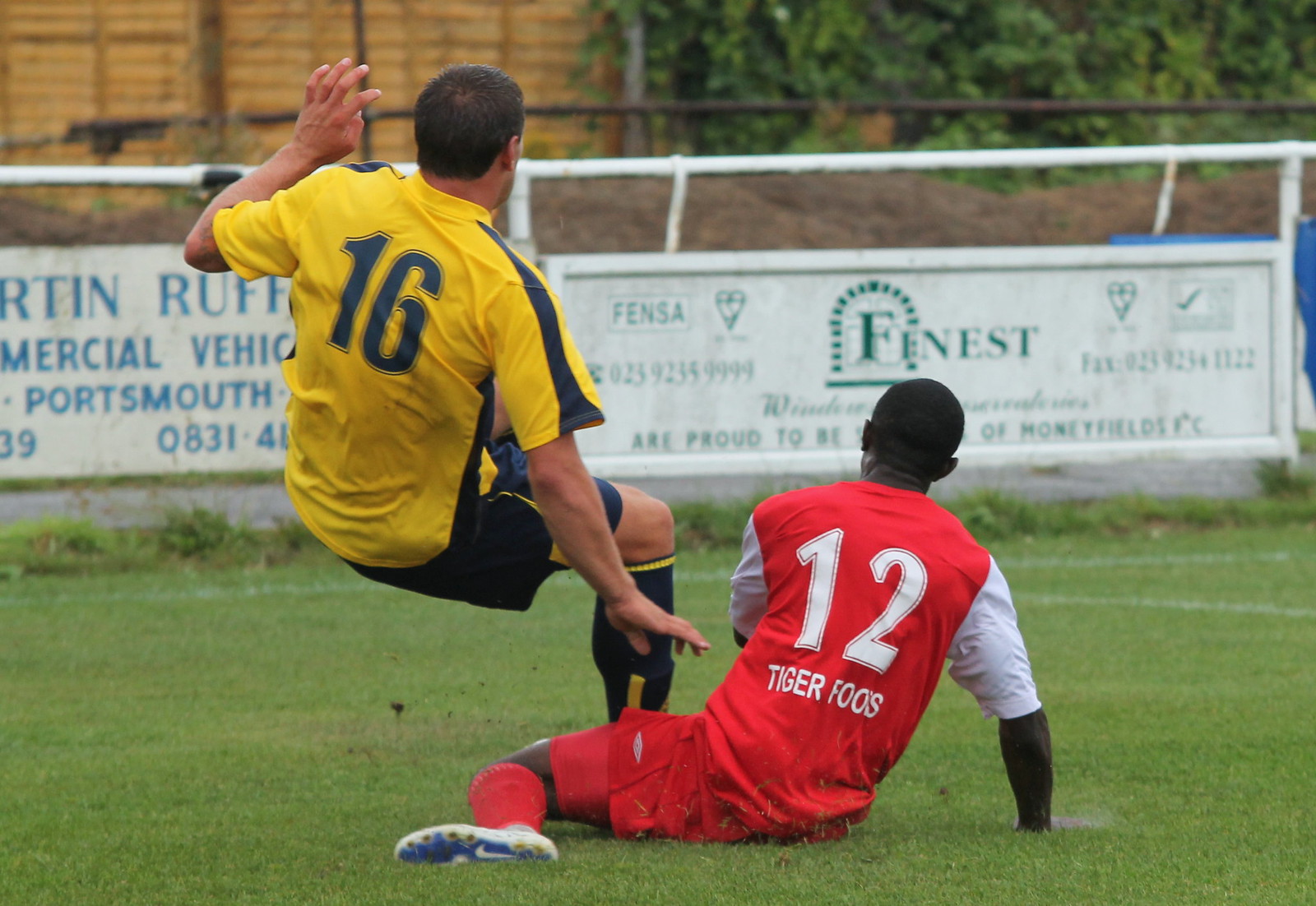In this vibrant outdoor scene, two male soccer players are captured in mid-action on a grassy field. To the left, one player is clad in a dynamic yellow jersey with blue shorts and matching socks, each adorned with a yellow stripe. His jersey displays the number 16 in dark blue as he leaps into the air, mid-jump with arms flailing to regain balance. Opposite him, a player dressed in a red and white jersey with the name "Tiger Foos" and the number 12 in bold white letters, along with matching red shorts and socks, is closer to the ground, suggesting he might have tripped his opponent. His right hand touches the ground, and his left arm is raised to stabilize himself. The backdrop features a white banner lined with green sponsor logos and a forest beyond, underscoring the bright day and adding to the dynamic tension of what seems to be a fierce mid-field collision, even in the absence of a visible soccer ball.